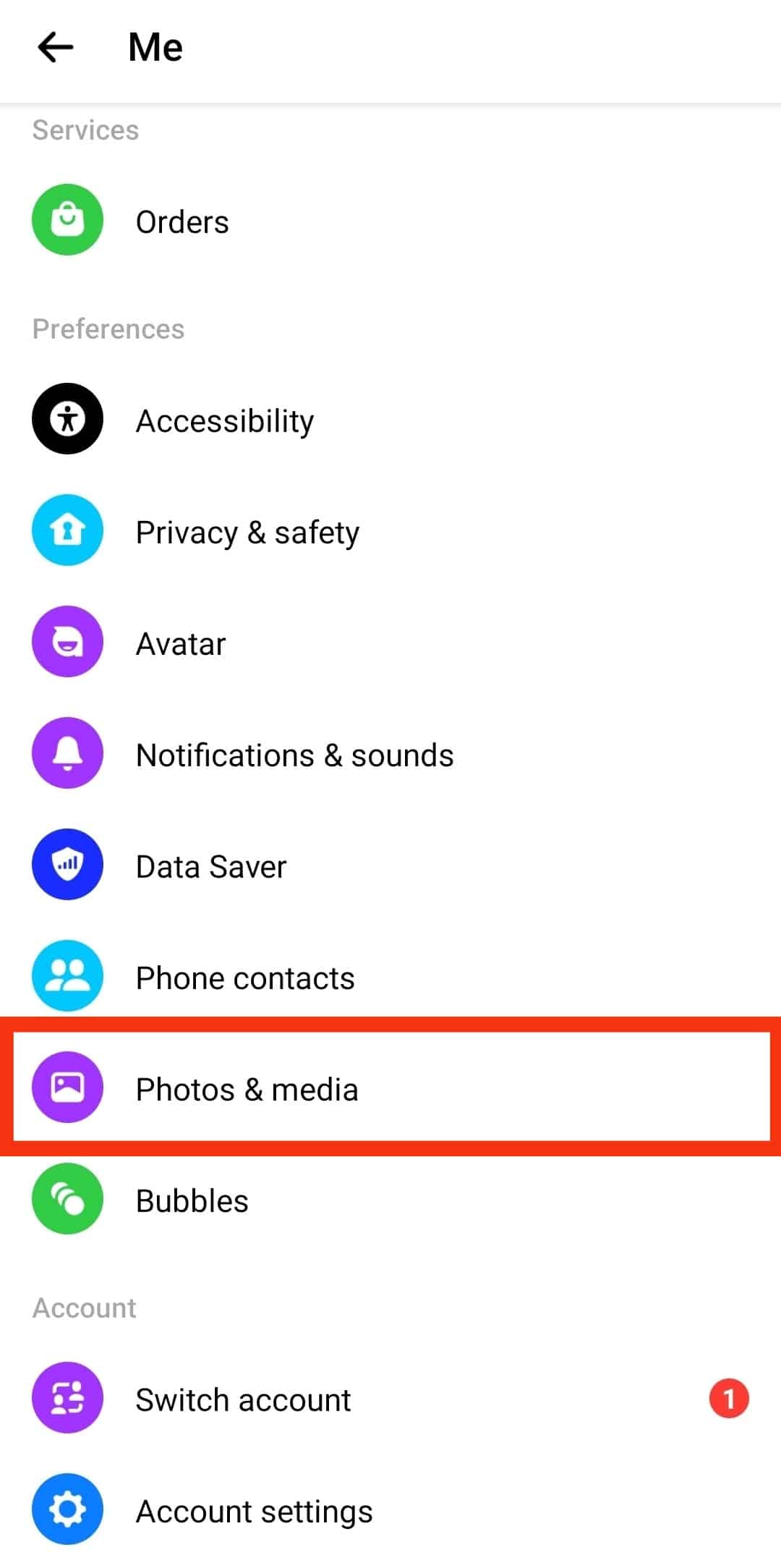This image is a screenshot showcasing the profile settings on a website or application. At the very top, there's a navigation indicator labeled "Me" with an arrow pointing left. Below that, several settings categories are listed:

1. **Services**: Accompanied by a green oval with the word "Orders."
2. **Preferences**: Marked with a black oval featuring a star icon and labeled "Accessibility."
3. **Privacy and Safety**: Denoted by a blue oval with a lock icon.
4. **Avatar**: Represented by a purple circle with an emoticon-like icon.
5. **Notifications and Sounds**: Indicated by another purple circle but with a bell icon.
6. **Data Saver**: Shown with a blue oval containing an emblem resembling a Wi-Fi signal strength icon.
7. **Phone Contacts**: Labeled with a light blue oval housing an icon of two head-and-shoulder figures.
8. **Photos and Media**: Highlighted by a purple oval with a files icon, and this option is currently selected, indicated by a large red rectangle surrounding it.
9. **Bubbles**: Displayed with a green oval, though its exact function is unclear—possibly related to pop-up notifications for incoming contacts.

The screenshot also includes an "Account" section, which features:

- **Switch Account**: Marked by a purple oval and accompanied by a red oval containing the number "1," likely indicating a notification or available account to switch to.
- **Account Settings**: Represented by a blue oval with a white gear icon.

Overall, the image provides a comprehensive view of various customizable settings within a user’s profile on the website or app.